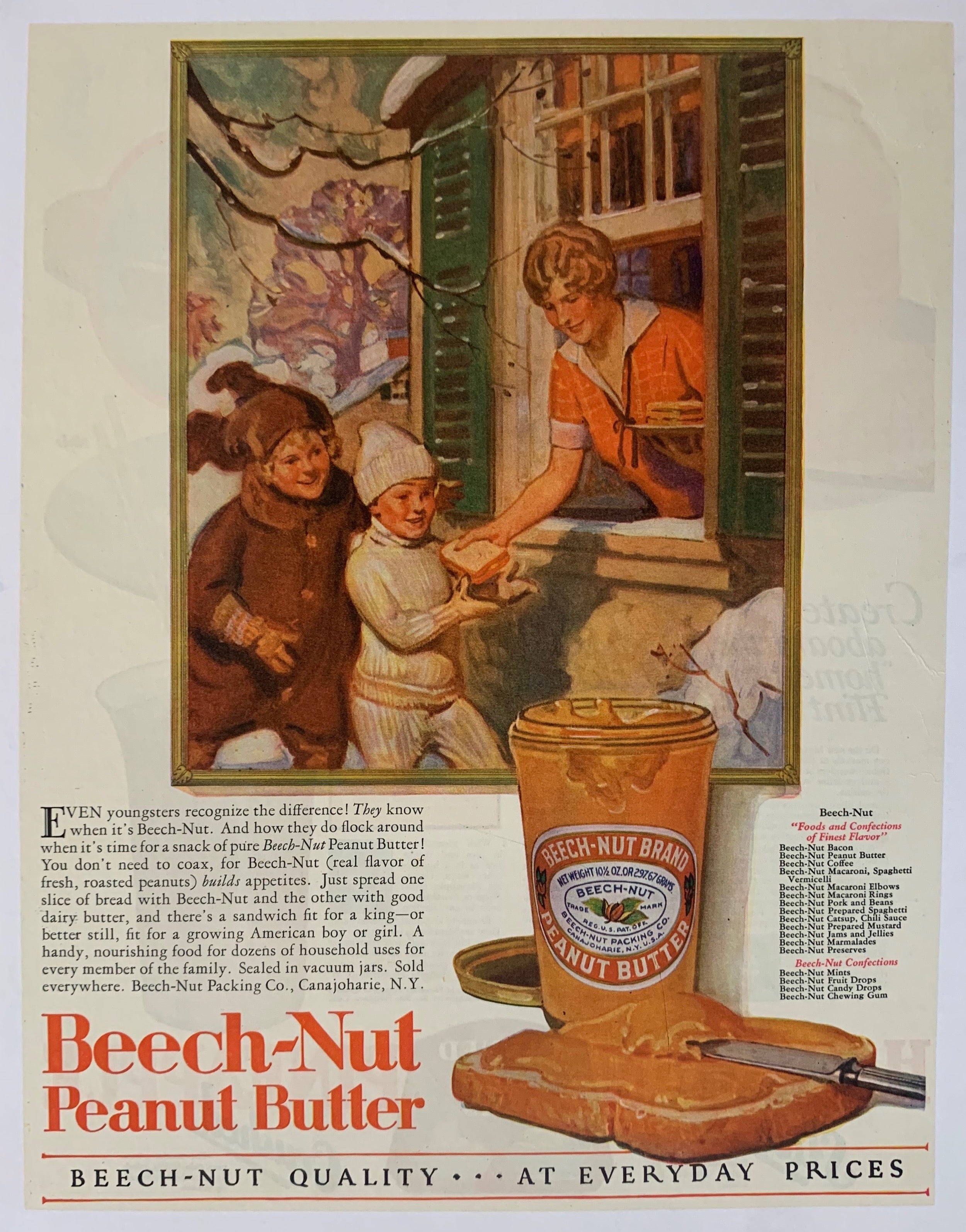This vintage magazine advertisement promotes Beech Nut Peanut Butter. Dominating the top portion, a vivid painting illustrates a winter scene with snowflakes gently falling. Two children, dressed in warm winter clothes, eagerly stand outside a house. Their mother, wearing a red shirt, leans out of a window, handing a freshly made peanut butter sandwich to one of the kids. Below the painting, a detailed paragraph extols the virtues of Beech Nut Peanut Butter. To the left of this text, the words "Beech Nut Peanut Butter" are prominently displayed in red font. On the right, a graphic showcases a jar of Beech Nut Peanut Butter, accompanied by a knife spreading the creamy spread on a piece of bread. At the very bottom of the page, the phrase "Beech Nut quality at everyday prices" is written in black text, emphasizing the affordability and high quality of the product.